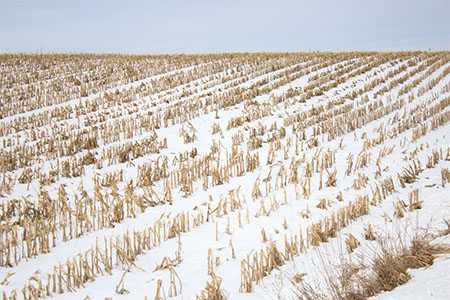The photograph captures a wintery farmland scene, dominated by rows of desolate, brown plants that appear dry and lifeless, likely remnants from a recent harvest. The field is meticulously organized with approximately 35 to 50 rows stretching diagonally from the bottom left to the top right, creating an impression of endlessness. The plants, resembling single stalks, rise sparsely from a landscape that alternates between patches of dirt and dead, yellowed grass. The sky above is a mix of gray and white, contributing to the overall dull and muted color palette of the image. The horizon line is faintly visible, marked by a hazy blend of blue and white clouds, further emphasizing the cold and barren atmosphere of the scene.